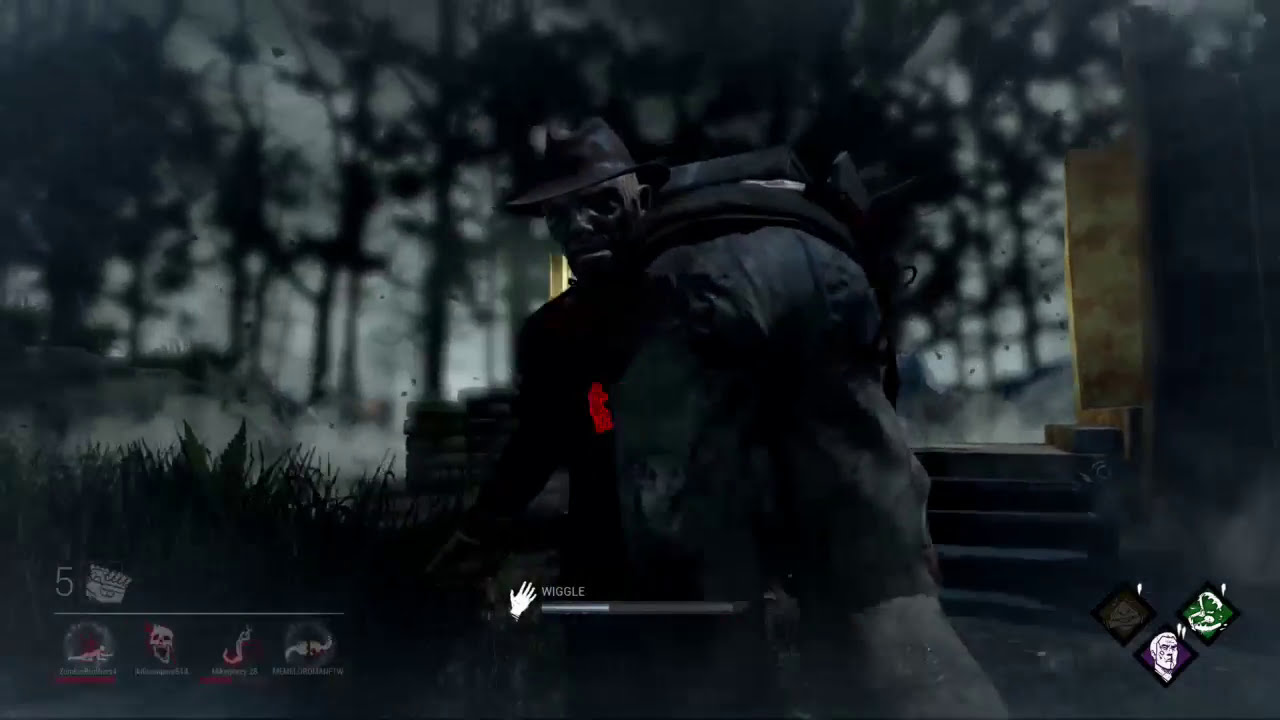In this dark and moody image, likely taken from a video game, a central figure stands facing the viewer. The character, silhouetted against a light gray sky littered with nearly black trees, wears a black fedora and has an eerie, almost skull-like face. His black attire blends into the shadowy scene, but a small red splotch is noticeable on his chest. His right hand is extended downwards, and he appears to be carrying another figure, draped in black pants and a vest, over his left shoulder. This secondary figure has long, black hair and seems more creature-like, potentially a zombie. At the bottom of the screenshot, on the left side, there’s a number "5" accompanied by several indistinct icons including one resembling a snake and another like a skull face. In the middle, the word "WIGGLE" appears above a white hand icon, which may denote some interactive element, perhaps a timeline bar beneath it. The right side of the screen also hosts various icons, including sideways triangles and a small image of a white face encased in a purple square. The entire setting, enhanced by tall trees, grass, and a few steps bordered by bricks and leafy plants, evokes an atmosphere of eerie desolation.